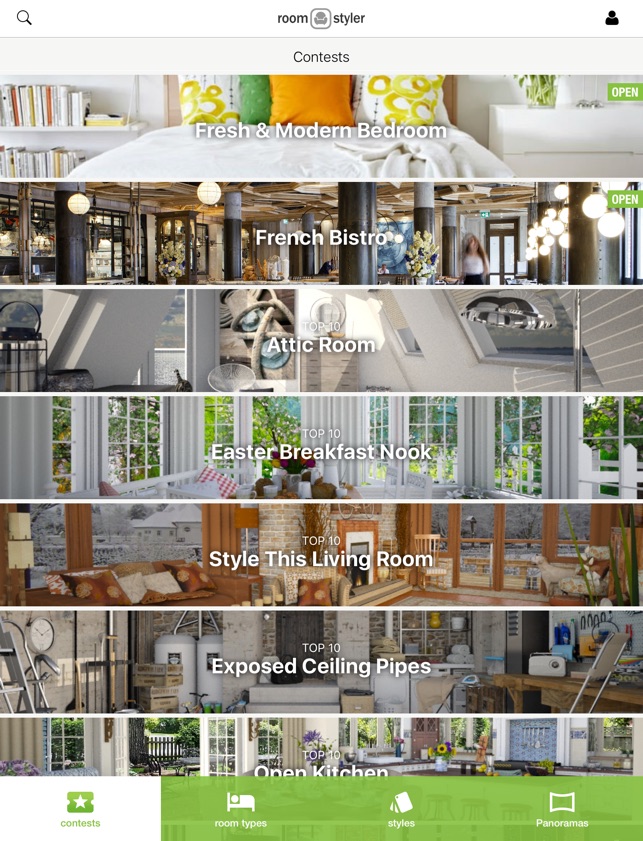The image showcases a web interface for a design application called "Room Styler." At the top, the title "Room Styler" is prominently displayed, with the word "Room" on the left, a couch icon in the middle, and "Styler" on the right. Directly beneath the title, there's a section labeled "Contest," which is divided into various design categories.

These categories include:
- **Fresh and Modern Bedroom:** Featuring minimalistic white sheets and simple solid colors, with a bookshelf positioned on the left side.
- **French Bistro**
- **Attic Room**
- **Easter Breakfast Nook**
- **Exposed Ceiling Pipes and Open Kitchen**

The layout suggests that users can enter these contests and see the top 10 designs in each category. Towards the bottom right of the interface, there's a prominent "Contest" button marked with an icon resembling a ticket with a star on it. Other options available at the bottom include "Room Types," represented by a bed icon, "Style," indicated by swatches, and "Panoramas," symbolized by a squashed rectangle.

At the top left corner, there is a search function, and on the far top right, a login option marked by a small black figure icon. This platform appears to offer both contest participation and design inspiration, serving as a useful tool for those interested in remodeling and interior design, akin to the style seen on HGTV.